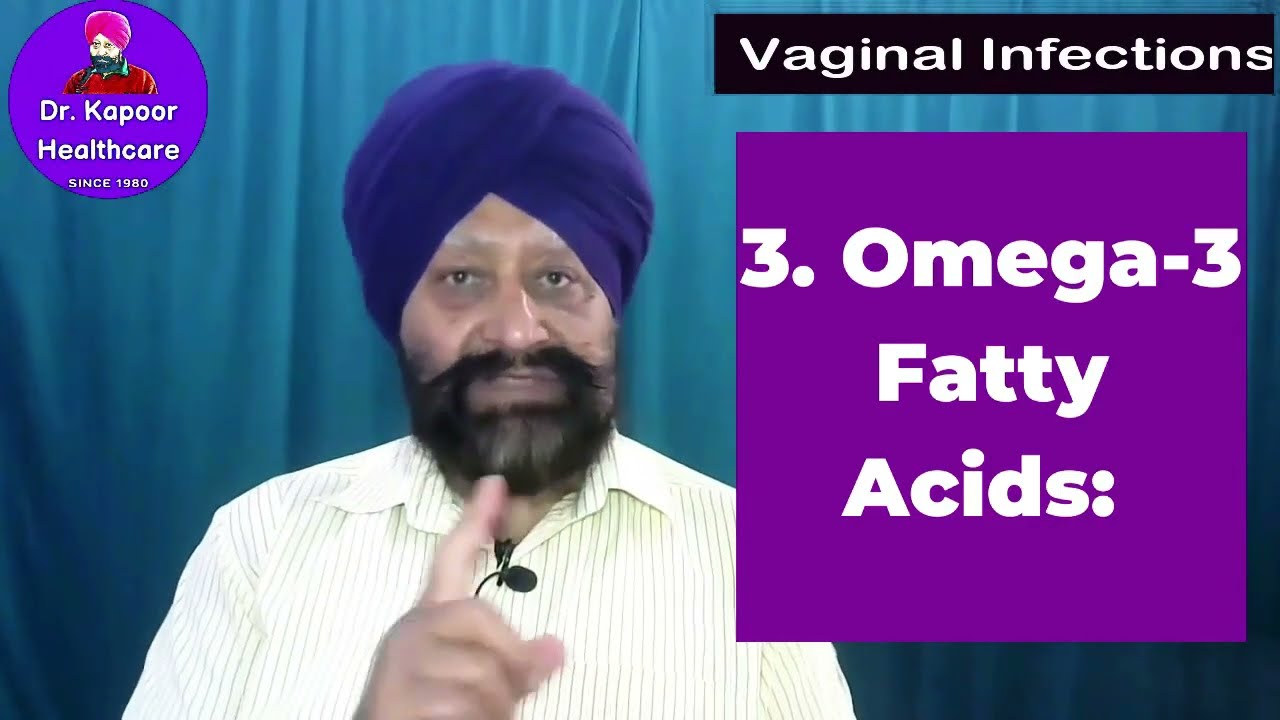The image appears to be a screenshot from a video or advertisement featuring health information. The background consists of medium-dark blue curtains with visible ripples and creases, confirming the fabric material. In the center, a man of Middle Eastern appearance is seen, wearing a dark purple turban, a white button-down shirt with thin vertical black stripes, and a black mustache and beard. He has a small black microphone clipped to the center of his neckline, beneath his chin. He looks directly at the camera and raises his right hand, with his pointer finger extended upwards as if to indicate the number one.

In the upper left-hand corner of the image, there is a digitally rendered purple square that includes a cartoon image of the man. Below this graphic, in white text, it reads, "Dr. Kapoor Healthcare, since 1980." On the upper right-hand corner, there is a horizontal black rectangle with white text that states "vaginal infections." Below this, a large purple square with white writing displays the text "3. omega-3 fatty acids."